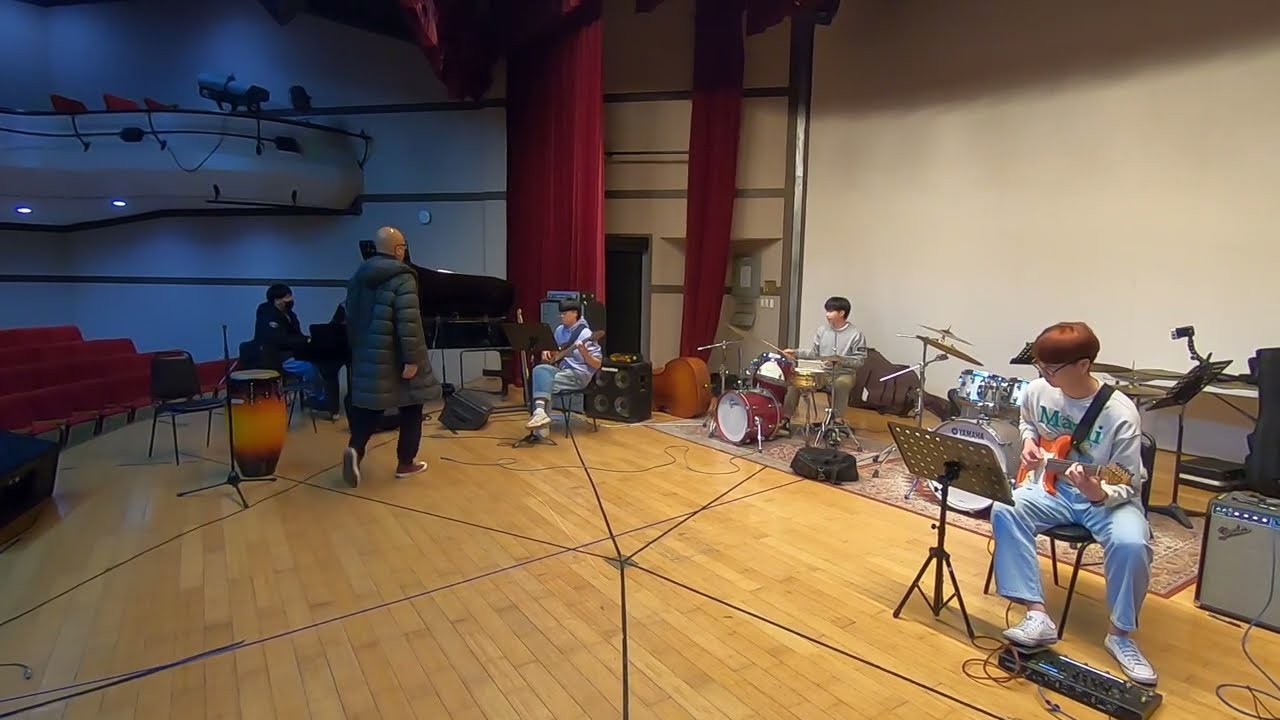In this photograph, a group of young boys, likely middle school or early high school age, are practicing their musical instruments on a large stage in an auditorium. The boys, who sport similar bowl cuts with one wearing glasses, are seated at music stands reading sheet music. One boy with orange-dyed hair, dressed in a white shirt, light blue jeans, and white sneakers, is playing an orange electric guitar with a black strap. Another boy, also dressed in casual attire, is seated further back, strumming a guitar. Toward the center is a boy playing drums, wearing khaki pants and a gray sweatshirt. The stage is characterized by a giant white banner behind them, hardwood flooring, scattered musical instruments, and empty seating, creating an impression of a rehearsal setting. A bald man in a coat, presumably their teacher, walks in front of them, monitoring their practice session. The array of stage lights and the absence of an audience further emphasize that the boys are preparing for a future performance.